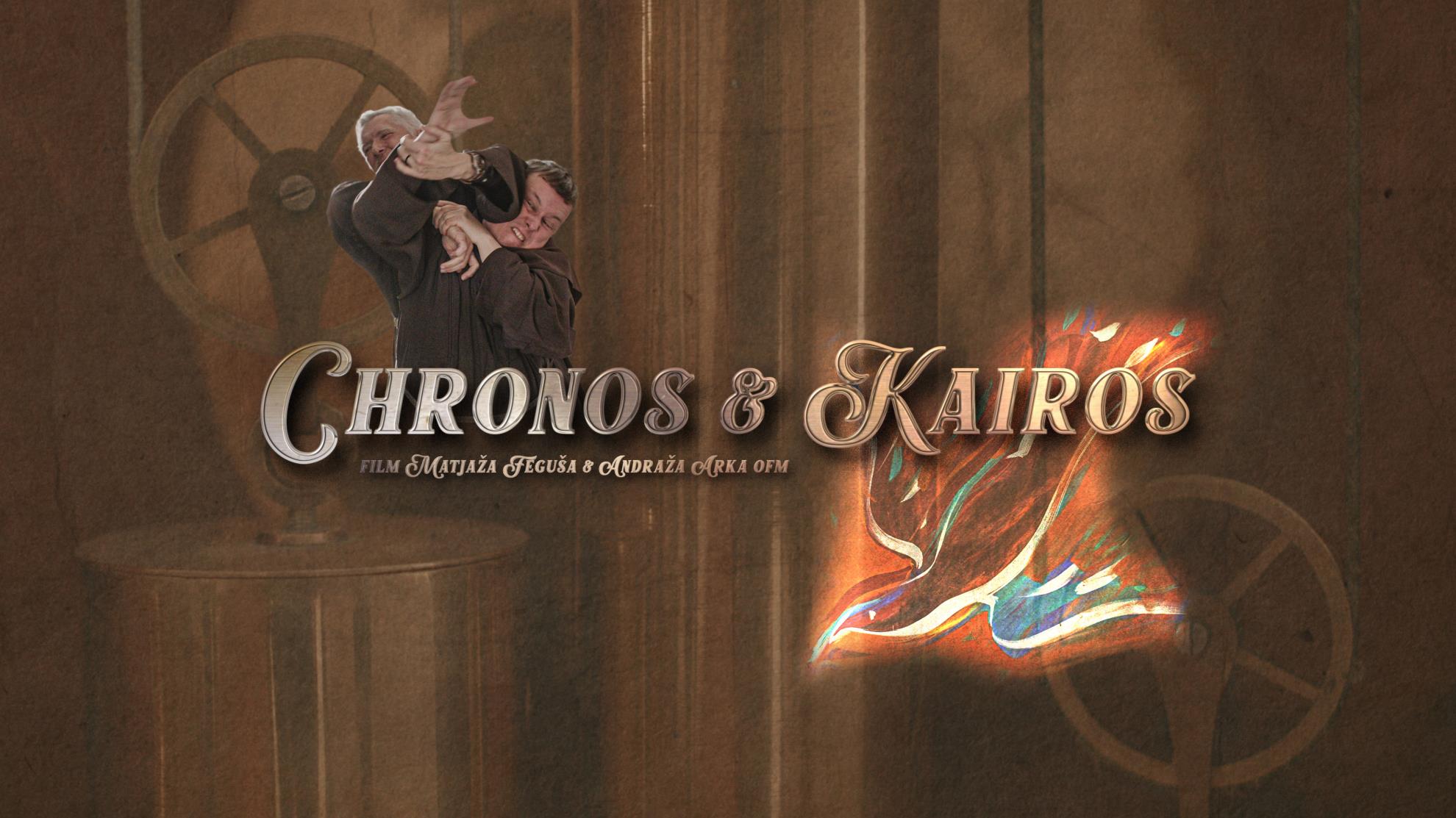The image is a rectangular composition, with a primary focal point on two individuals engaged in a struggle. The older, white-haired man and the younger, brown-haired man, both clad in brown robes, are depicted gripping each other's wrists and shoulders, with one man's elbow in the other's face. These figures are crisp and striking against a faded, steampunk-inspired background featuring bronze metal circles, ropes, and wheels atop metal cylinders, rendered in a brownish-gold monochrome.

Central to the image, bold white text reads "Kronos & Kairos," with the ampersand prominently joining the names. Beneath this title, in smaller font, various non-English words appear, likely indicating a film title: "Film Majaza, Fegusa, and Andraza, Arca, OFM." Directly below the name Kairos, there's an abstract, colorful rainbow bird, possibly representing a phoenix, adding a vivid splash of color to the otherwise muted background. The overall scene blends elements of conflict, time, and mythology in a visually intriguing design.